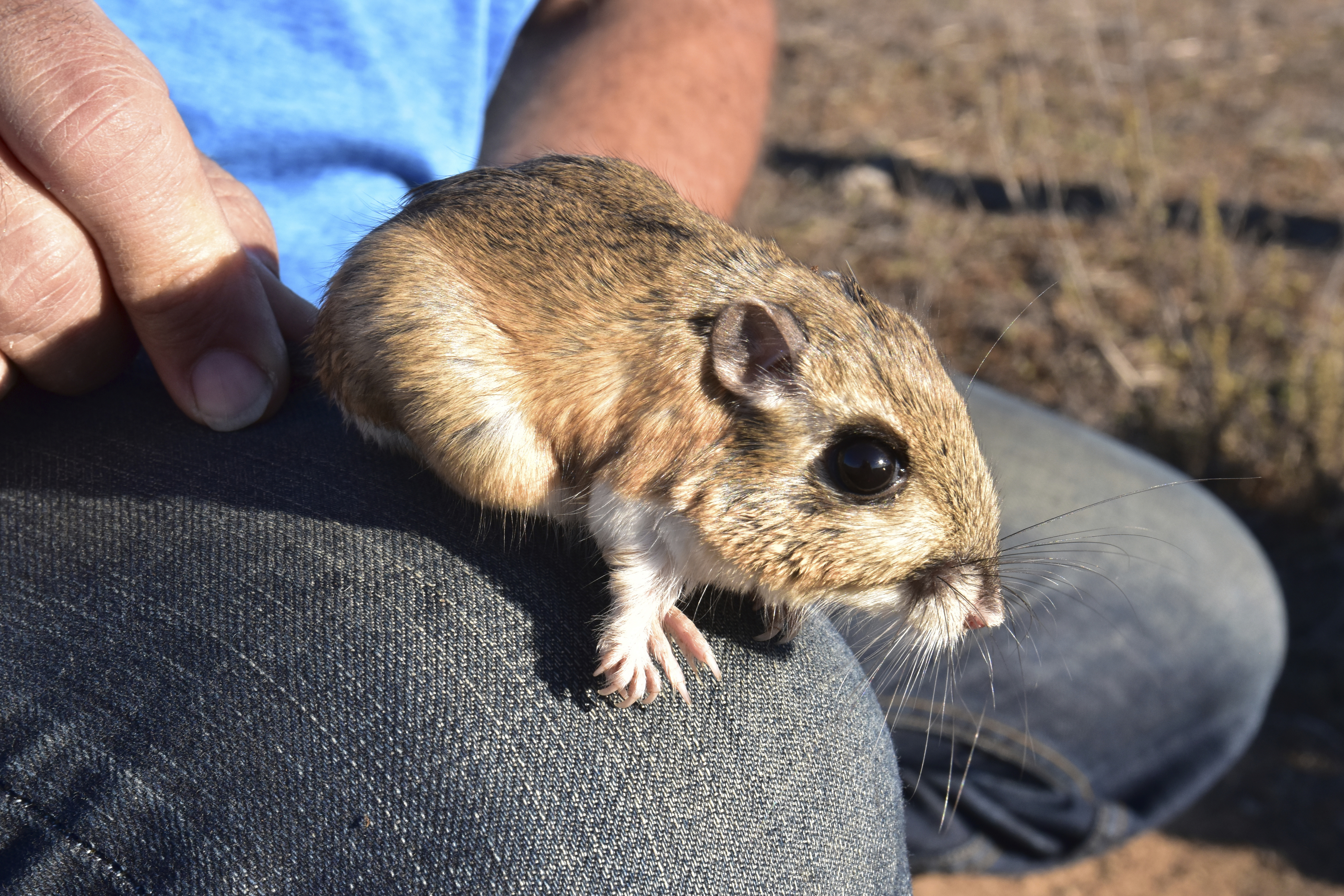In this image, a small creature, possibly a chipmunk or sugar glider, is sitting on the knee of a man's pants, which appear to be blackish-blue. The man is wearing a light blue shirt and has Caucasian skin, with his left arm and hand partially visible behind the animal. The creature itself has a distinctive appearance with a short body, a large head, very large round black eyes, small grayish ears, and a tipped nose. Its body is predominantly brown with traces of black and lighter brown, and it has a white underbody. The creature's feet appear webbed and its claws are long and pinkish. In the blurred background, there is a dirt field with sparse patches of grass and another person squatting or kneeling, wearing jeans.